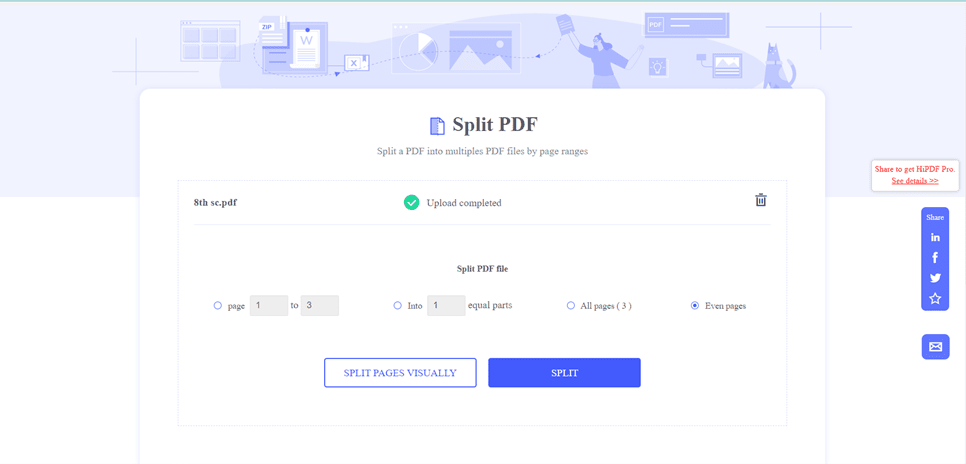"Image depicting the process of splitting a PDF using software tools. A user interface showcases options for dividing a PDF by specified page ranges. The completed task is summarized, indicating that the file has been successfully uploaded and split. The user chose to split the PDF into individual pages, specifically from pages one to three. The selected mode is 'Even Pages Only', highlighting tools for visual page split confirmation."